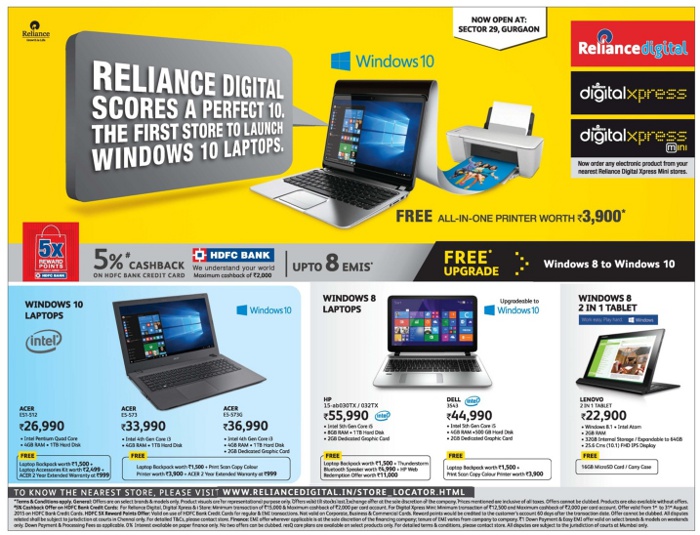Caption:
Reliance Digital proudly announces the opening of its newest store at Sector 29, Gurgaon. With a striking promotional banner featuring a vibrant yellow rectangle, the store has become the first to launch Windows 10 laptops. The banner showcases several key details:

- A prominent red square highlighting the Reliance Digital logo.
- Two black squares, one of which includes the "Digital Express" branding.
- An exciting offer of a free all-in-one printer valued at $3,900*.
- A distinctive currency symbol and a picture of a bag indicating financial incentives.
- A promotion of 5 TOMs reward points in blue and 5% cashback on offers, specifically in collaboration with HDFC Bank.
- Financing options available with up to 8 EMIs.
- Details about a free upgrade from Windows 8 to Windows 10.

The banner also displays three images: the first featuring a laptop with price tags for Windows 10 laptops from Acer, starting at ₹26,990 and another model priced at ₹33,990. This grand opening combines technology, finance, and exclusive rewards, making it an irresistible destination for tech enthusiasts.